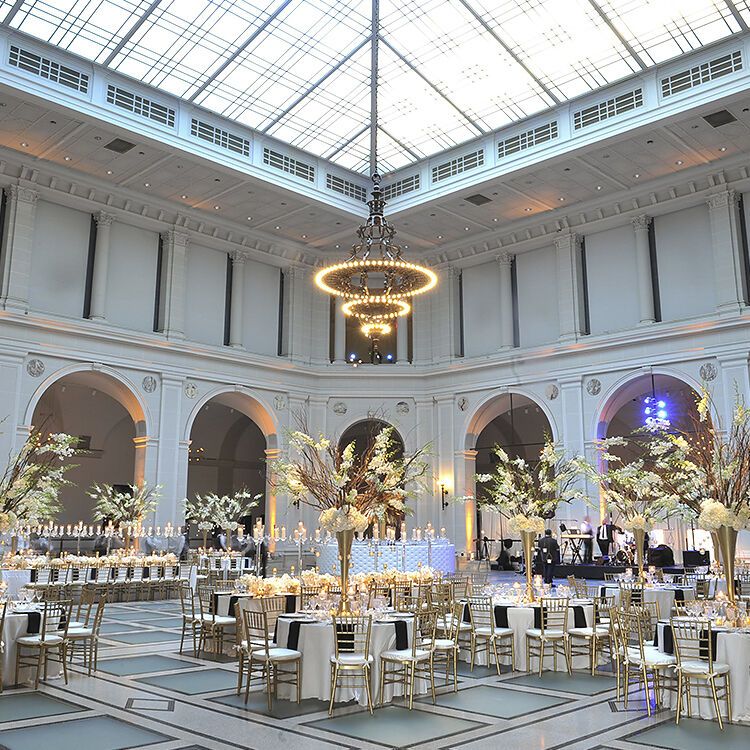This image captures an opulent ballroom, possibly being prepared for a wedding, characterized by its very tall glass ceilings that allow an abundance of natural light to filter through. Dominating the center of the room is a grand, three-tiered chandelier with circular arrays of light bulbs that increase in size from bottom to top. The ballroom is dotted with numerous circular tables elegantly dressed in white tablecloths, each surrounded by gold-hued chairs fitted with white cushions.

The tables feature striking, tall centerpieces resembling trees, set in slender, gold-colored vases adorned with white flowers. Surrounding the room are large, white archways—five in total—that lead to various sections of the ballroom, along with towering columns that add a regal touch to the space. The floor is a mosaic of blue and white tiles that complement the overall lavish decor.

On the right-hand side of the image, a small stage is visible, occupied by men in suits with musical instruments, indicating an upcoming performance. Meanwhile, on the left side, preparations for a buffet can be seen with dishes arranged on a white-draped table. Overall, every aspect of the space speaks to its grandeur and meticulous preparation for a significant event.